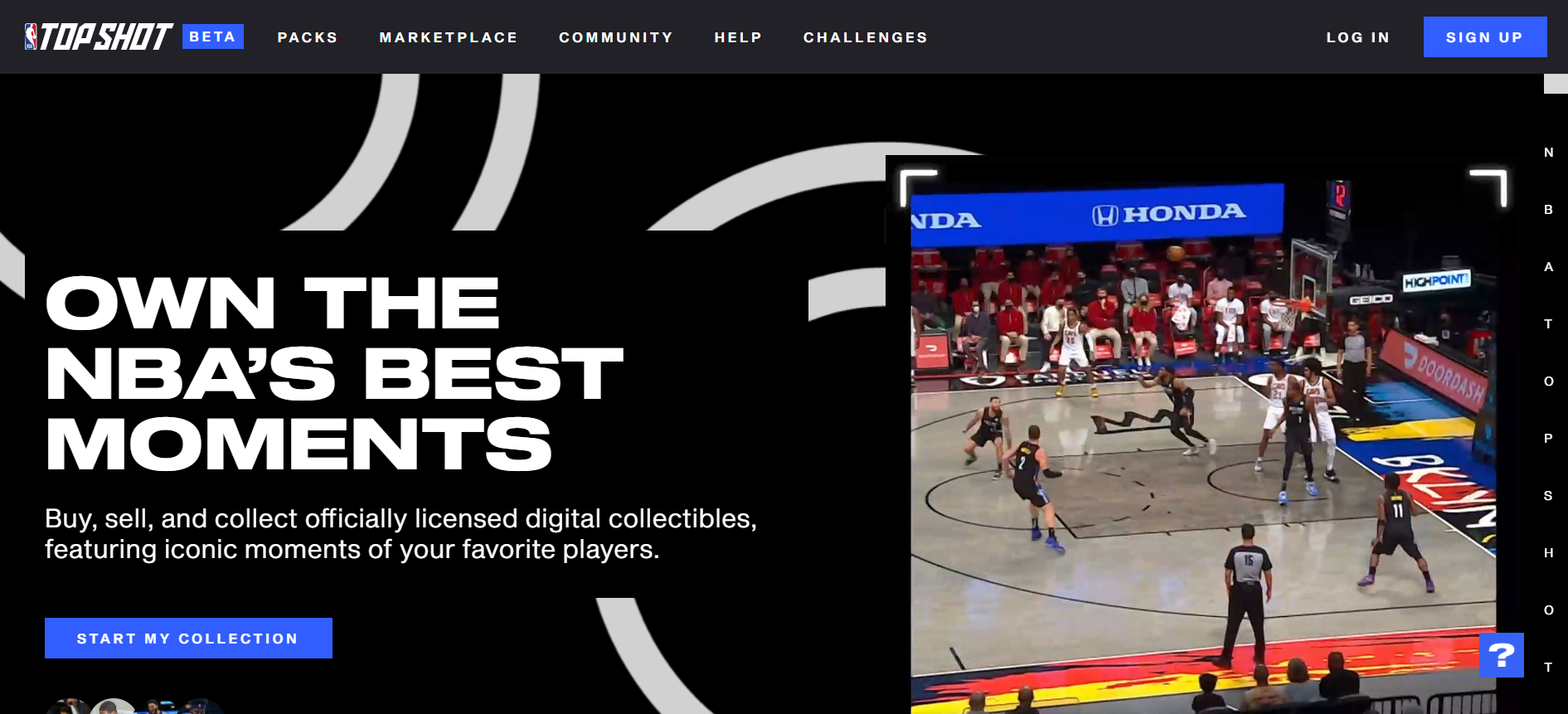Screenshot of the NBA Top Shot website interface showcasing their digital collectibles platform. At the top of the screen, the NBA logo and “Top Shot” are displayed prominently alongside a “Beta” label in a blue box. Navigation options including "Packs," "Marketplace," "Community," "Help," and "Challenges" are lined up in white text. On the right side, options for "Login" and "Sign Up" are present, with the latter in a rectangular box.

Centrally, large white text reads, "Own the NBA's Best Moments," followed by smaller text detailing the platform's offering: "Buy, Sell, and Collect Officially Licensed Digital Collectibles Featuring Iconic Moments of Your Favorite Players." Beneath this, a clickable blue rectangular button labeled "Start My Collection" invites users to begin their digital collection.

In the background, white swooshes overlay a vivid image of an active basketball game. Advertising banners for Honda, DoorDash, Geico, High Point, and a possible reference to "BKLYN" are visible above the spectators. A blue question mark icon is located at the bottom of the image. The basketball court is occupied by around seven or eight players, though their diverse attire suggests they may not be professional athletes.